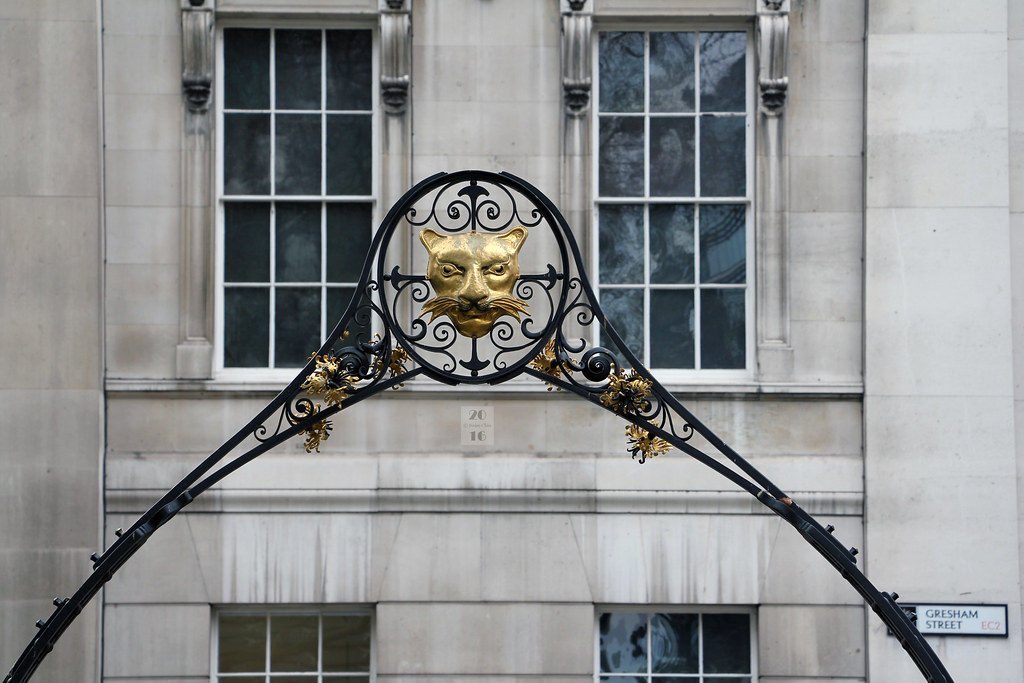The photograph captures a close-up view of a large city building with a stucco façade, tinged in light gray pastel, set against a somewhat cloudy sky. Dominating the scene are two prominent picture windows on either side, each approximately six feet tall, segmented into twelve panes with decorative framing. The top panes feature small, circular ornaments with etched faces, creating a refined architectural detail. In the lower section of the photo, additional half-windows are visible, maintaining the paneled style but truncated at the base.

At the heart of the image stands an intricate metal archway. This ornate structure is crafted from wrought iron with a central circular element displaying a gold-colored lion's face, possibly a female lion due to the absence of a mane but with distinguishable whiskers. The archway's decorative features extend along its edges with a mix of arrows pointing in cardinal directions and smaller gold ornaments flanking the lion's face. Notably, a small white placard sign reading 'Gresham Street' is visible near the bottom right of the window arrangement, adding a touch of urban context to the elegant architectural focal point.